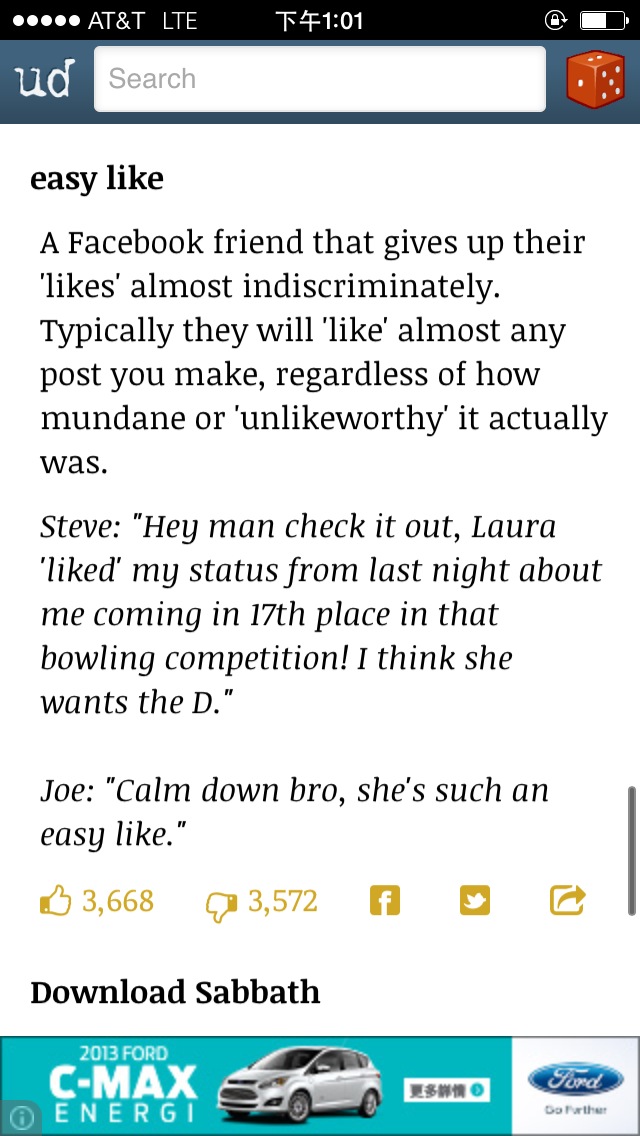This is a detailed screenshot of a smartphone app or web page. At the top, a black header features the text "AT&T LTE" on the right, five white dots on the left, some Chinese characters in the center accompanied by the number "101," and a battery indicator at about 50-60% on the far right. Just below, a white search bar is displayed with the letters "UD" on the left and a red die icon on the right.

Further down, against a white background, a heading in bold blue and black text reads "EASY LIKE". The accompanying paragraph defines an "Easy Like" as a Facebook friend who indiscriminately likes posts, regardless of their significance. Below this description are italicized dialogue lines:
"Steve: Hey man, check it out, Laura liked my status from last night about me coming in 17th place in that bowling competition. I think she wants the D."
"Joe: Calm down, bro. She's such an easy like."

The image also includes social interaction stats and icons as follows: a gold thumbs-up icon with the number "3,668", a thumbs-down icon with the number "3,572", followed by icons for Facebook, Twitter, and a forwarding arrow. At the bottom, the text "Download Sabbath" appears above a banner ad for the 2013 Ford C-MAX Energi vehicle.